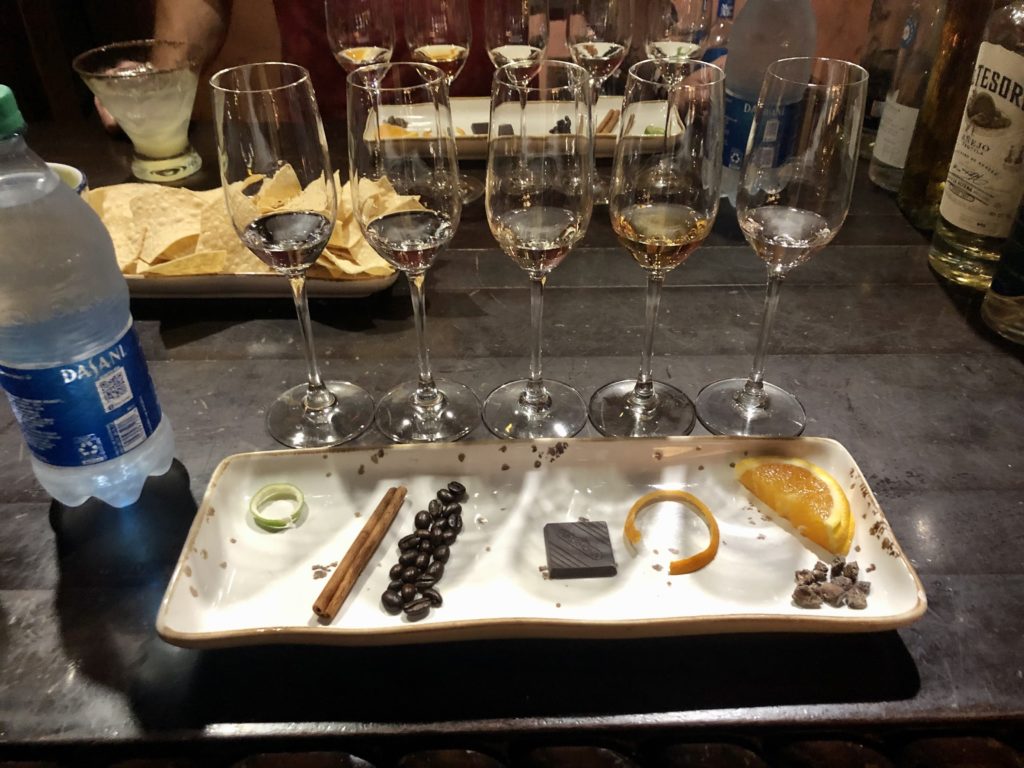The photograph captures an elegantly set dark brown tabletop, featuring a detailed arrangement indicative of a recent toast. Central to the composition is a rectangular ceramic tray laden with various leftovers. This tray holds two long cinnamon sticks, a few black coffee beans scattered on a smear of cream or frosting, a piece of rectangular, embossed chocolate, a few citrus peels, and a slice of orange. The tray is accentuated by chocolate shavings.

Positioned directly behind the tray are five tall wine flutes, each containing a small amount of liquid, hinting at a recent celebration. To the left of the tray sits an unopened bottle of Dasani water. Further back on the left side of the table, a small platter of tortilla chips is visible, accompanied by a slightly yellowish drink in a small glass that could be interpreted as a margarita. In the background, partly obscured, is a patron with an arm extending into the frame. On the far right, a wine bottle labeled “TSOR” stands among other liqueur bottles, adding to the refined yet casual ambiance that could represent either a bar setting or an intimate gathering at a friend's home.